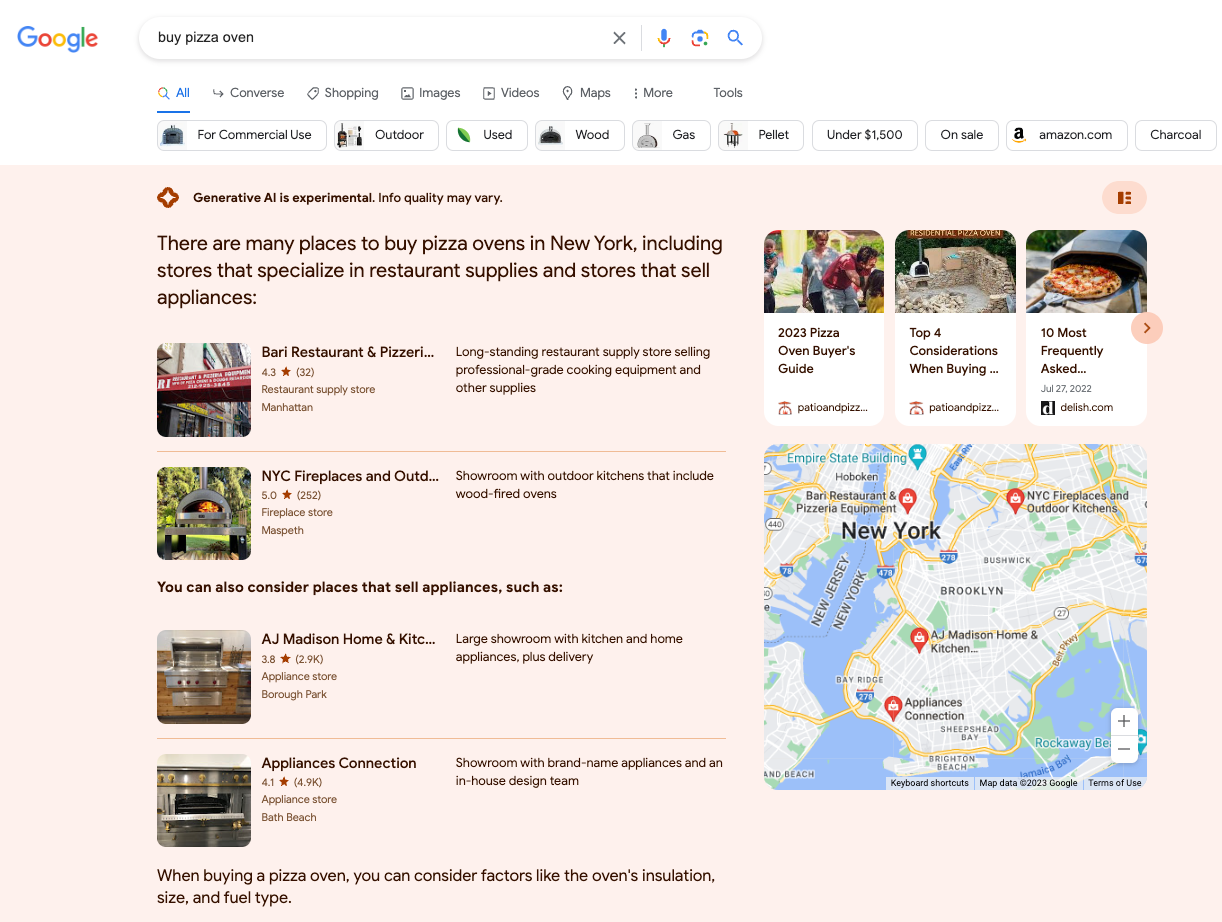This image showcases a Google search result page. At the top, the iconic colorful Google logo is prominently displayed. Below it, the search query entered is "buy pizza oven," accompanied by an "X" to clear the search, a colorful microphone icon for voice search, a camera icon for visual search, and a blue magnifying glass icon to initiate the search.

The search results page features various filters for refining the search, including categories like "All," "Converse," "Shopping," "Images," "Videos," "Maps," "More," and "Tools." Additional options for narrowing down the search include "commercial use," "outdoor," "used," "wood," "gas pellet," "under 1,500," "on sale," "Amazon.com," and "charcoal."

At the top of the search results, a message states, "Generative AI is experimental, info quality may vary." The initial search results provide information on where to buy pizza ovens in New York. It mentions different types of stores, including those specializing in restaurant supplies and those that sell various appliances.

Highlighted results include "Bari Restaurant and Pizzeria," described as a long-standing store offering professional-grade cooking equipment and other supplies. Another featured option is "NYC Fireplaces," which has a showroom with outdoor kitchen setups that include wood-fired ovens. Additional recommendations suggest appliance sellers like "A.J. Madison Home and Kitchen," known for their large showroom with home delivery, and "Appliances Connection," which offers a showroom featuring brand-name appliances and an in-house design team.

The search results also emphasize important factors to consider when buying a pizza oven, such as the oven's instructions, size, and fuel type. A map at the bottom displays the locations of these stores, marked with red pinpoints in various neighborhoods, and provides links to their respective websites.